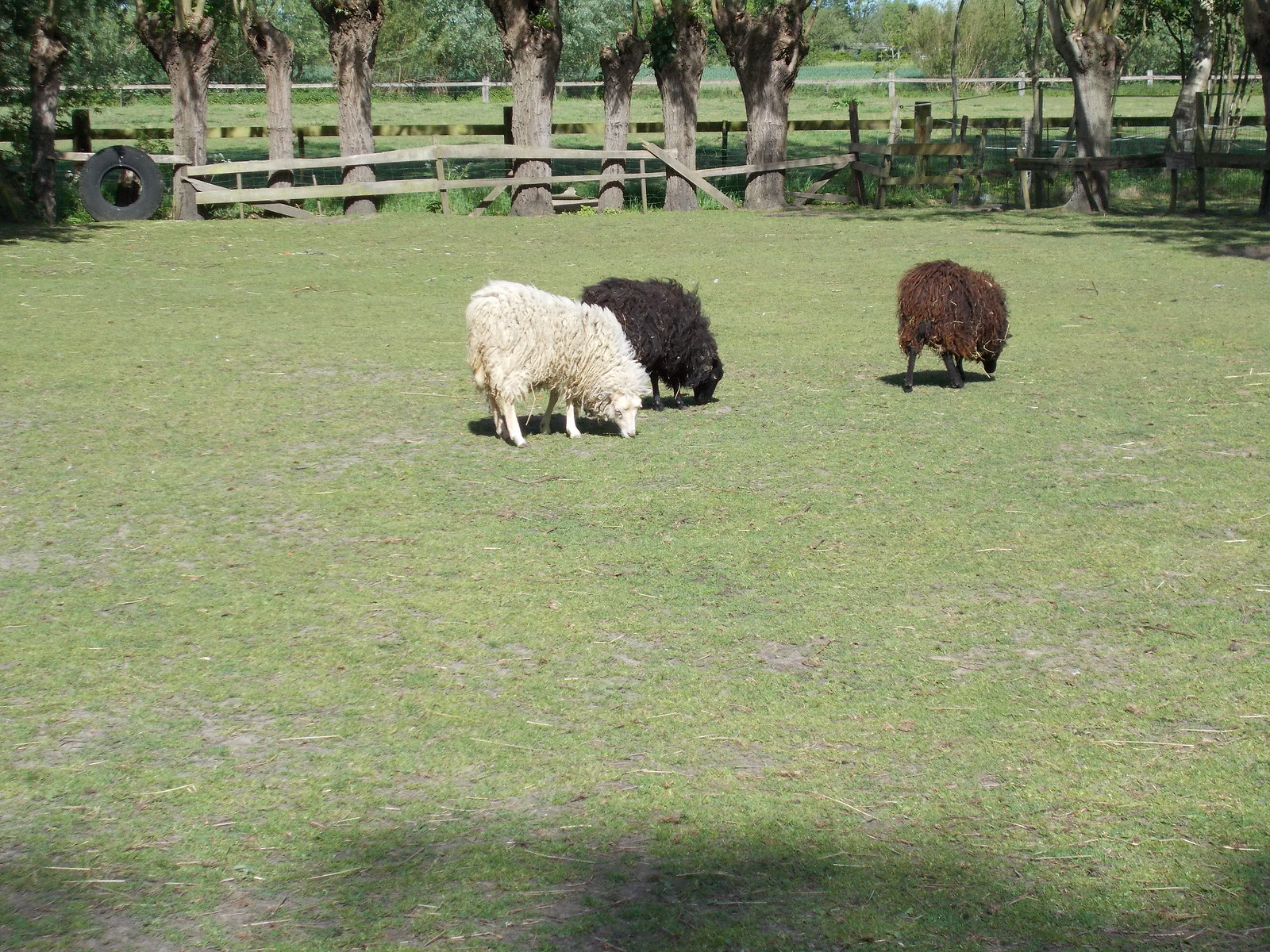This photograph captures a picturesque, outdoor ranch setting on a sunny day. In the foreground, three sheep—one white, one black, and one brown—grazing on short, neatly trimmed grass. The field is enclosed by wooden slat fencing that runs between and around a number of trees, approximately ten of which are discernible. Several enclosed areas with wooden fences can be seen, indicating it's likely a ranch. A black spare tire is positioned in the upper left-hand corner of the scene. Shadows from the trees create cool patches along the bottom edge of the image, which overall has a squared shape. Beyond the main field, another fence and a secondary tree line extend into the background, providing depth and a lush, pastoral atmosphere.